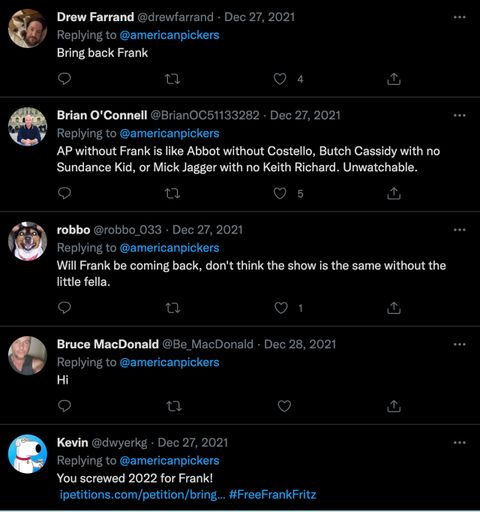A black screen displaying several left-justified comments, each accompanied by a profile icon, forms the focus of this image. The comments are as follows:

1. Drew Farland (@DrewFarland) – December 27, 2021:
   "Replying to American Pickers: Bring back Frank."

2. Brian O'Connell (@BrianOC511332A2) – December 27, 2021:
   "Replying to American Pickers: AP without Frank is like Abbott without Costello, Butch Cassidy without the Sundance Kid, or Mick Jagger without Keith Richards. Unthinkable."

3. Robbo (@Robbo_033) – December 27, 2021:
   "Replying to American Pickers: Will Frank be coming back? Don't think the show is the same without the little fella."

4. Bruce McDonald (@TheBe_McDonald) – December 28, 2021:
   "Replying to American Pickers: Hi."

5. Kevin (@DWYERKG) – December 27, 2021:
   "Replying to American Pickers: You screwed 2024 for Frank. I Petitions.com/petition for is that, bring... #FreeFrankFritz."

The comments reflect the users' reactions to the absence of Frank Fritz from the show "American Pickers," emphasizing their desire for his return and the perceived impact of his absence on the show's quality.